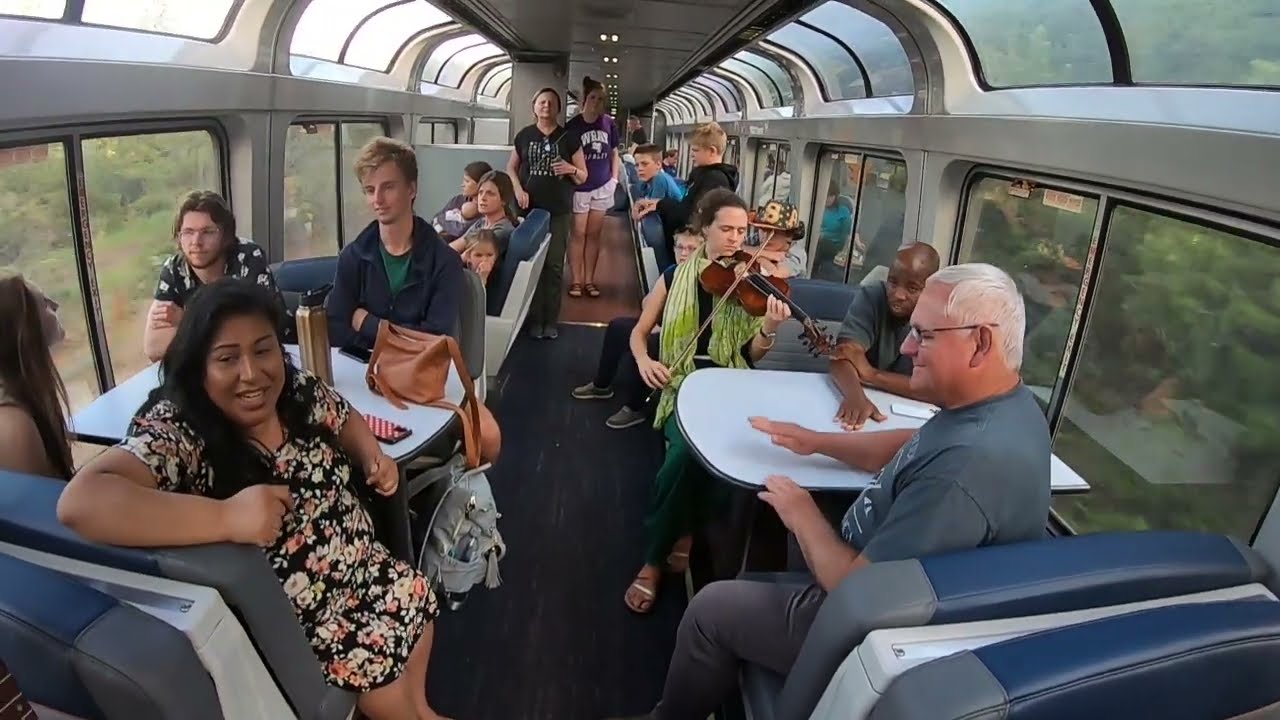The photograph captures the interior of a passenger train car, viewed from one end looking down its length. Large glass windows, both on the side walls and the curved ceiling, offer an illuminated view of the lush greenery and trees outside, giving the impression of an aerial perspective. The interior is well-lit, with white fixtures and a mix of dark blue and navy blue seating featuring gray accents. The flooring transitions from dark blue carpeting to what appears to be brown hardwood.

Inside, the train car is bustling with around two dozen passengers. They are seated at white tables in navy blue seats, some facing forward, others turned in various directions. Several people are standing in the aisle. On the right, a fair-skinned, heavyset man with white hair and glasses, dressed in a gray t-shirt and jeans, looks toward the aisle. Opposite him sits a dark-skinned woman with long black hair, wearing a black and white floral print dress, turning her head toward the camera.

A woman in a lime green scarf plays the violin, adding a musical ambiance. Most passengers, absorbed in conversations or enjoying the scenic view, seem to be listening to her music. The setting is lively, with people standing around the aisle, including a woman in a purple top and white shorts. The colors in the image range from gray, dark blue, light green, white, dark green, silver, brown, to purple, and there is no text or signage visible. The overall scene conveys a moment of leisurely travel through a scenic route during the daytime.